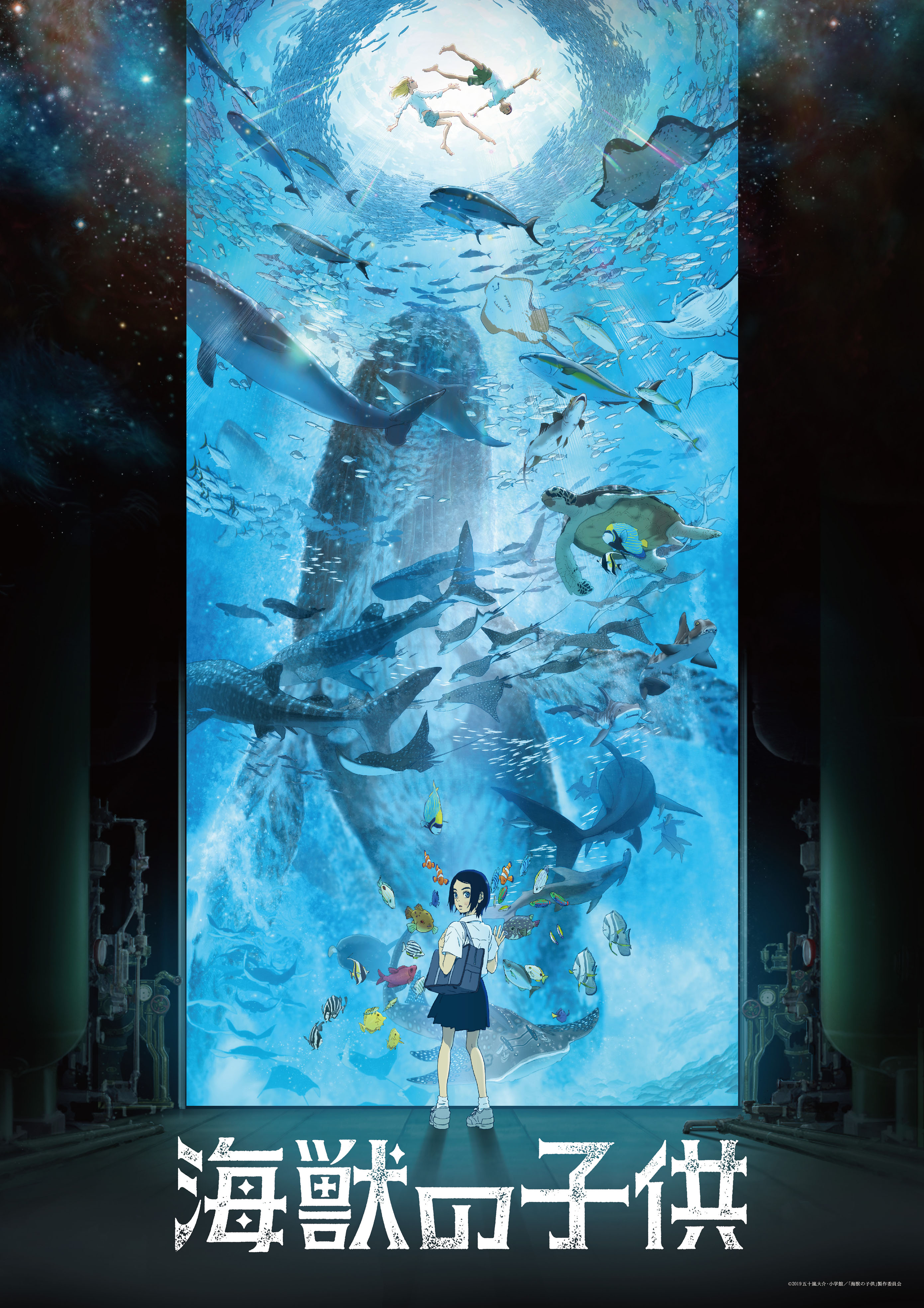This image features a detailed cartoon illustration, reminiscent of a Japanese movie poster. Central to the scene is a large aquarium filled with diverse marine life, including a gigantic blue whale, several sharks, a green turtle, and a variety of colorful fish such as yellow, striped, and pink species. Two individuals are seen swimming at the top of the aquarium, seemingly out of place.

In the foreground, a young girl wearing a short skirt, gray shoes, and carrying a blue shoulder bag turns to look toward the viewer, positioned as if she is part of the scene. Behind her, the aquarium background extends into what appears to be a stylized galaxy of stars. The entire illustration is overlaid with Asian lettering, suggesting the title and details of the movie, which remain unreadable. The ambiance of the image is whimsical and vibrant, combining elements of aquatic life with a touch of cosmic wonder.